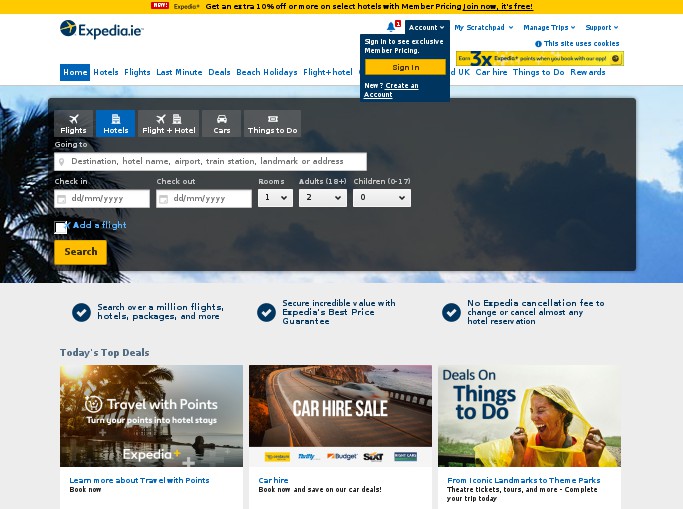This web page for Expedia features a vibrant gold ribbon at the top, prominently displaying a special offer in dark blue text that reads: "Expedia: Get an extra 10% off or more on select hotels with member pricing." The text "Join now, it's free!" is underlined, encouraging users to sign up. Directly below this banner, on a white background in the upper left-hand corner, the word "Expedia.ie" appears in bright blue text, accompanied by a navy blue circle with a gold airplane icon.

To the right, a notification bell icon shows pending notifications, followed by options labeled "My Scratchpad", "Manage Trips", and "Support" in bright blue ink. The "Account" section is highlighted against a navy blue background and urges users to "Sign in to see exclusive member pricing," with a gold-colored "Sign In" button featuring navy blue text.

Below this section, the main image showcases a serene blue sky dotted with a few white clouds and the top of a swaying palm tree. Superimposed over this background, a gray box contains a navigation bar with five smaller tabs: "Flights", "Hotels", "Flight+Hotel", "Cars", and "Things to Do". The "Hotels" tab is currently highlighted.

Centered below the tabs is a search bar labeled "Going to", inviting users to input their "Destination, hotel name, airport, train station, landmark, or address". Additional fields are provided for "Check-in" and "Check-out" dates (month, day, and time), "Number of rooms", "Adults", and "Children". To finalize the search, a gold "Search" button stands out, ready to be clicked.